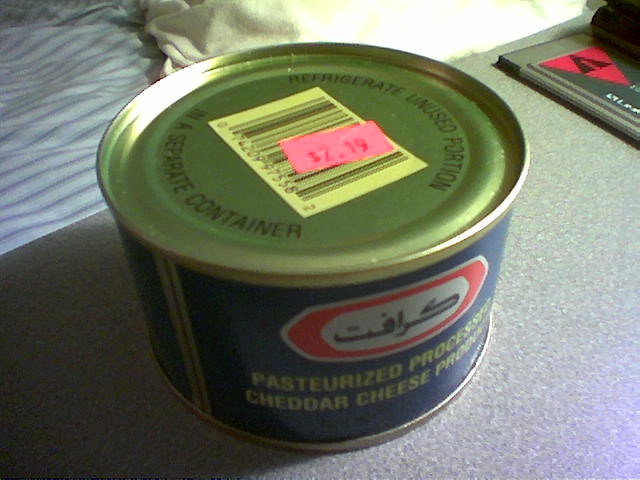A slightly blurred photograph captures a small canister of food, akin to the size of a typical tuna can but with a rounder and slightly taller profile. The can's top is a metallic gold, with an inscription advising to "refrigerate unused portion in a separate container." Dominating the front, a blue label features gold lettering that reads "Pasteurized Processed Cheddar Cheese Product." Adjacent to this, a blue and white logo with Arabic script adds a touch of cultural distinction. Atop the can, a pink price tag is prominently displayed, indicating a cost of $2.19. The image's lack of sharpness suggests it may have been taken with a lower-quality camera.